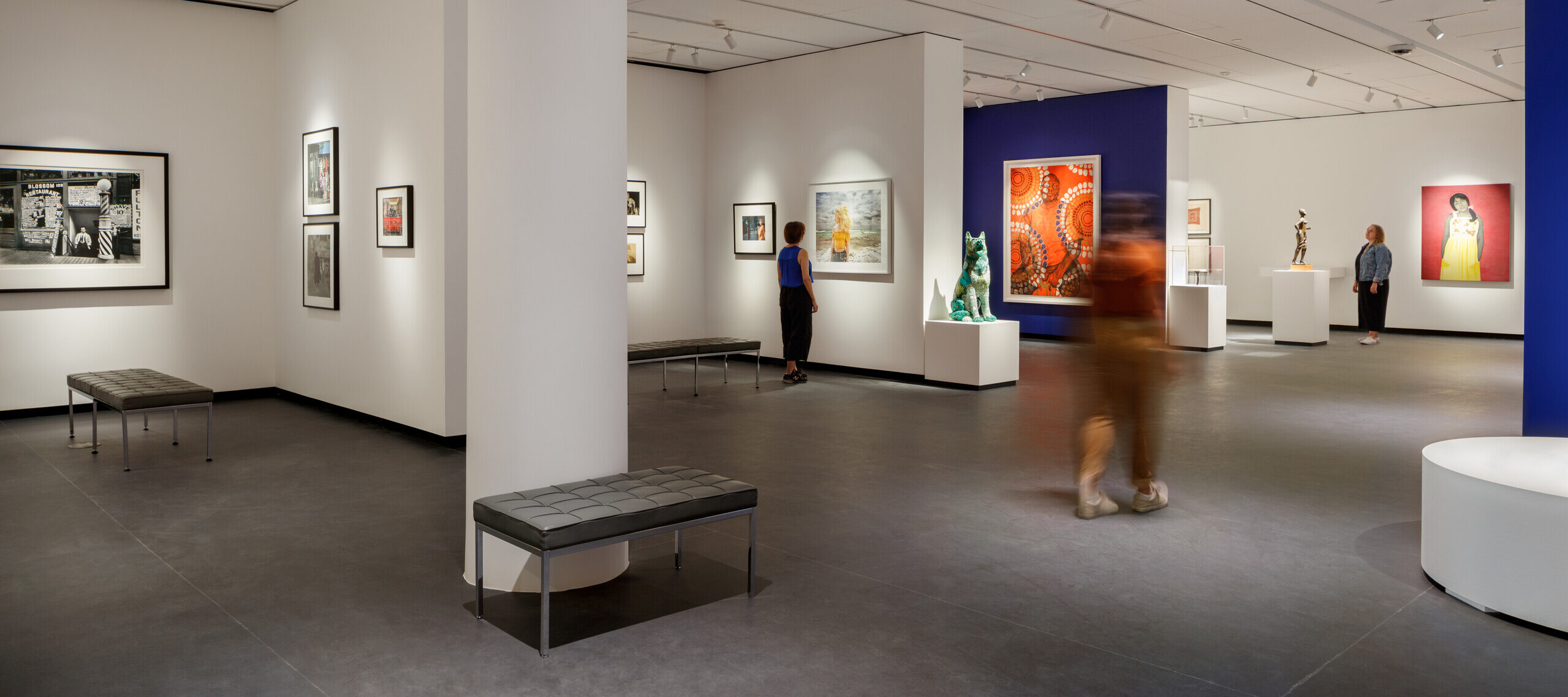The photograph captures the interior of a spacious art gallery with predominantly white walls interspersed with a distinct royal blue section. The gallery features multiple cubicles with framed black-and-white photographs and an array of other artworks. Notably, one wall showcases an abstract orange painting. The floor is uniformly gray, enhancing the minimalist aesthetic of the space. Visitors in the gallery are seen observing the art—one woman in a black skirt and denim jacket examines a bronze sculpture while another in a yellow top and black skirt studies a piece from a distance. In the center of the image, there is blurred motion of a passerby, adding a dynamic element to the otherwise static scene. Additionally, a small green sculpture of what seems to be a dog or wolf stands on a white pedestal. The arrangement includes occasional benches for visitors to sit and reflect on the art. The directional lighting highlights the artworks, creating a focused ambiance in this serene and contemplative environment.